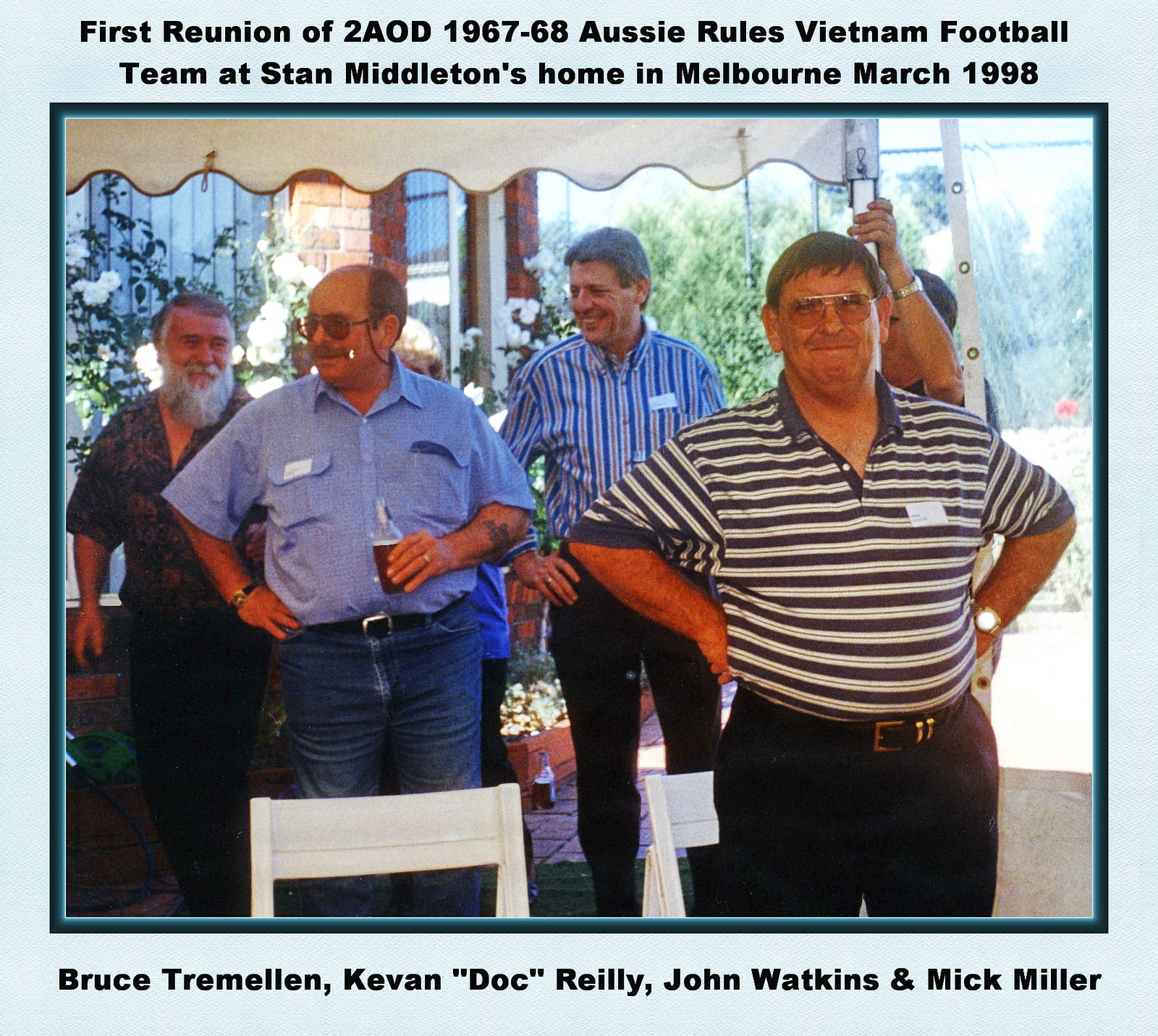In the image, five men are gathered under a white canopy among an array of white chairs, appearing to enjoy a reunion in a backyard setting with visible grass and trees. The man in the forefront, positioned to the right, sports dark brown hair, glasses, and a closed-mouth smile. He dons a collared shirt with blue and white stripes, sleeves reaching his elbows, black pants, and a white patch on his chest. His elbows are bent outward, hands resting on his ribs. Behind him, slightly to the left, stands another man with graying hair, wearing a shirt with blue, yellow, and white stripes and black pants, his head turned left, and one hand on his hip.

Adjacent to him, nearer to the front, a man in a solid light blue shirt grasps a bottle with brown liquid at stomach level. He has sunglasses, a balding receding hairline, blue jeans, and his other hand is placed on his hip. Farthest to the left, a man with a broad white beard and gray hair is visible. In the background, the white backs of chairs lead your eye to a building with brick columns, window panels, and a partly visible balcony with a wavy bottom ridge.

On the right edge of the scene, a hand wearing a gold watch holds onto a canopy support. Text above the group reads, "First reunion of two AOD, 1967 to 68, Aussie rules Vietnam football team at Stan Middleton's home in Melbourne, March, 1998." The bottom of the picture lists the names of four men, although five are visible in the image. The setting and attire suggest a relaxed, outdoor atmosphere where old friends have gathered to reminisce and celebrate their shared history.